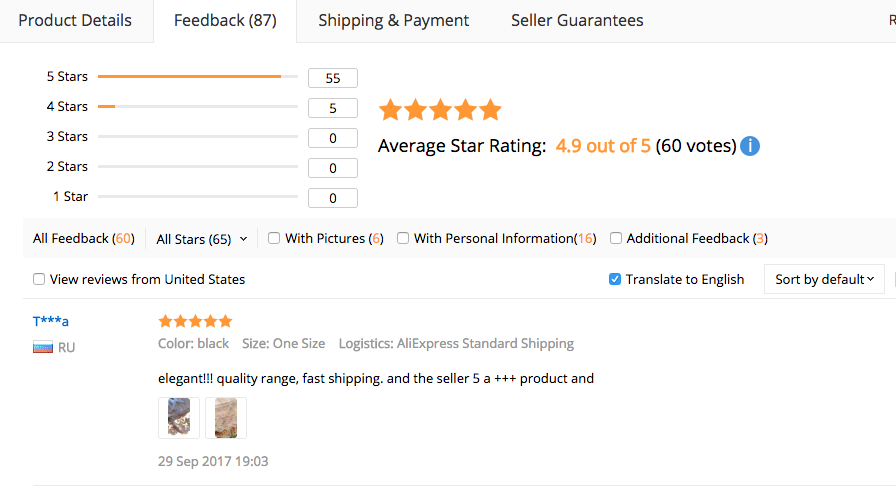This screenshot captures the review section of an Aliexpress product page. The website has a clean, white background with several navigation tabs at the top: Product Details, Feedback, Shipping & Payment, and Seller Guarantees, with the Feedback tab currently selected, displaying the number 87 in parentheses.

The feedback section contains user ratings for a product described as "Elegant Quality, Color: Black, One Size," with shipping handled through Aliexpress Standard Shipping. While the exact nature of the product is unspecified, the ratings distribution is prominently shown: 55 five-star ratings, 5 four-star ratings, and no three-star, two-star, or one-star ratings, leading to an impressive average rating of 4.9 out of 5 stars based on 60 reviews.

A 'Translate to English' button is checked, indicating that the page was originally in a foreign language — likely Russian, as evidenced by the "RU" and Russian flag icon next to the username in the lower left corner. This suggests the webpage was translated into English for accessibility.